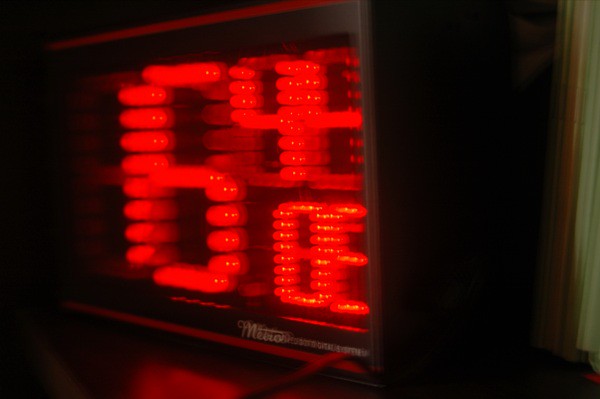This indoor color photograph is a close-up of a digital clock, captured from an angle that only reveals the right side of the clock while the left side remains obscured in darkness. The clock features a black box with an LED display that illuminates red numbers. The numbers appear distorted and blurred, likely due to low image quality, motion blur, and reflections on the screen. The display appears to be showing "1542" or possibly "1540," with an additional "8" or "E" in the lower right corner. The background is dark and the image is slightly out of focus, making it challenging to discern the exact numbers or whether it is indicating the time or another type of information. A subtle hint of green can be observed on the right edge of the photograph.